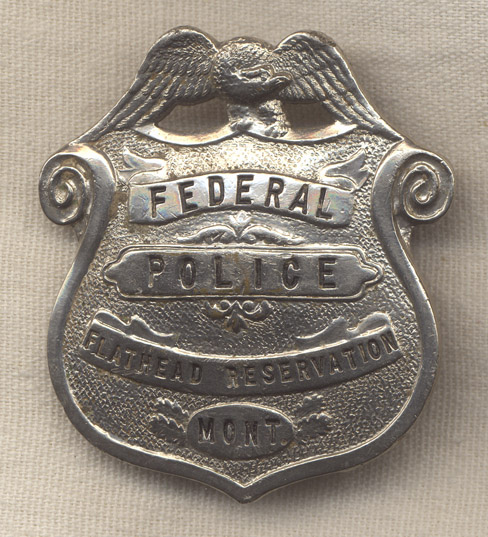The image features a tarnished silver police badge made from a shiny, metallic metal, likely steel or aluminum. The badge is shaped like a shield and prominently displays an eagle with spread wings at the top. Beneath the eagle, the badge reads "Federal Police, Flathead Reservation, MONT." The text is set against a raised rectangular background, using a font that appears to be sans-serif. The badge is adorned with engravings of leaf shapes and finely detailed borders. Notable is the badge's somewhat worn and rust-speckled appearance, adding character to its predominantly silver color. The badge is set against a light tan or grayish fabric backdrop.